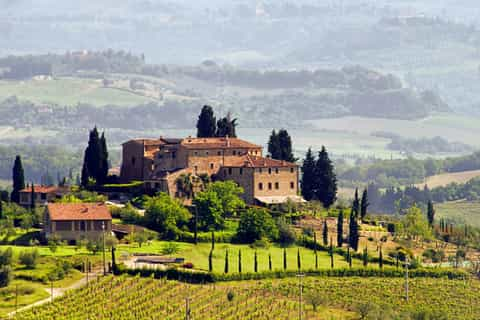The image depicts an expansive estate captured from an elevated position, possibly from a hilltop or even from an airplane. The scenery revealed is both picturesque and grand, with a sprawling chateau-like villa that exudes a Tuscan aesthetic. This large, beige mansion, standing about three or four stories tall, commands the foreground. The estate itself is composed of several large buildings or sections, with a possible gatehouse situated towards the front.

Surrounding the mansion is a meticulously manicured front lawn, accompanied by tall trees strategically placed on both the left and right sides. In the immediate foreground, you notice gardens or fields featuring row planting, potentially vineyards with grape vines, interspersed with posts from fencing. These cultivated lands extend into a hilly vista beyond the mansion, transitioning into vast agricultural fields and open grasslands.

A couple of smaller buildings can be seen towards the back left of the image, contributing to the estate's grandeur. The scene is further enriched with scattered trees and small pathways or roads that weave through the landscape. As you gaze further into the distance, the image becomes increasingly hazy, with tree lines demarcating various properties and wooded areas blending seamlessly with farming grounds. The overall impression is that of a serene, idyllic countryside estate framed by a balance of natural and cultivated beauty.